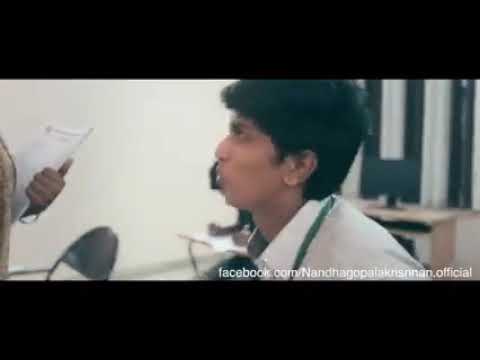The image appears to be a low-resolution, blurry screenshot clipped from a video, possibly originating from a Facebook page. It captures a classroom scene featuring a young man, likely of South Asian or Middle Eastern descent, seen from his left side profile. The young man has dark, poofy hair reminiscent of an Elvis style and tan skin. He is wearing a white collared shirt with a green-trimmed white sweater or a lanyard around his neck. The setting appears to be a classroom where the young man is engaging with a woman in front of him who is holding a stack of papers, suggesting a possible teacher-student interaction, potentially regarding a test result. The presence of other students behind him, one seated at a desk and another chair visible, reinforces the classroom environment. The image has black borders at the top and bottom, and in the bottom right corner, there is a URL: facebook.com/N-A-N-D-N-A-G-O-P-A-L-A-K-R-I-S-N-N-A-N.official.